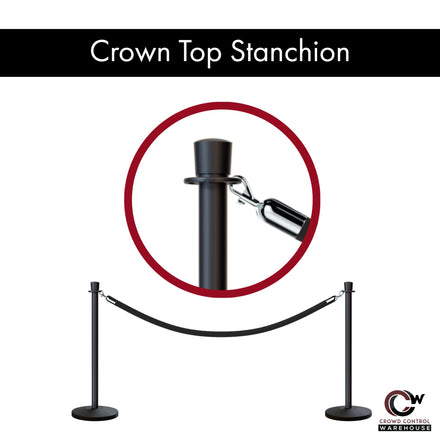This image prominently showcases a crown top stanchion, a component of a line divider often used in places like clubs or events to guide people. The stanchion is a black pole with a shiny metal hook which attaches to a red velvet rope, creating a barrier. The image is organized in a detailed, diagrammatic style typically seen in advertisements. A red-circled close-up focuses on the top part of the stanchion, revealing the white text label "Crown Top Stanchion" against a black rectangle. Below this zoomed-in section is an illustration of the full setup, with two poles connected by a rope in a typical red carpet or crowd control layout. The bottom right corner features a logo for Crowd Control Warehouse, with "warehouse" highlighted in black. The overall colors in the image are black, white, red, and silver, on a clean white background.